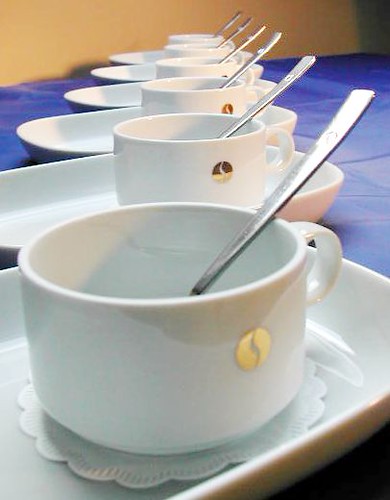This photograph captures a close-up arrangement of six white ceramic mugs, each delicately resting on white paper doilies within rectangular, slightly rounded dishes. The mugs, adorned with a gold circle featuring an S-like or lightning bolt design, align symmetrically in a diagonal row extending towards the image's background. Each mug contains a silver teaspoon, placed consistently with handles pointing to the right. The setup sits atop a distinct blue tablecloth, with a tan or golden wall providing a warm backdrop, suggesting a well-prepared setting, possibly for a buffet or a formal gathering.